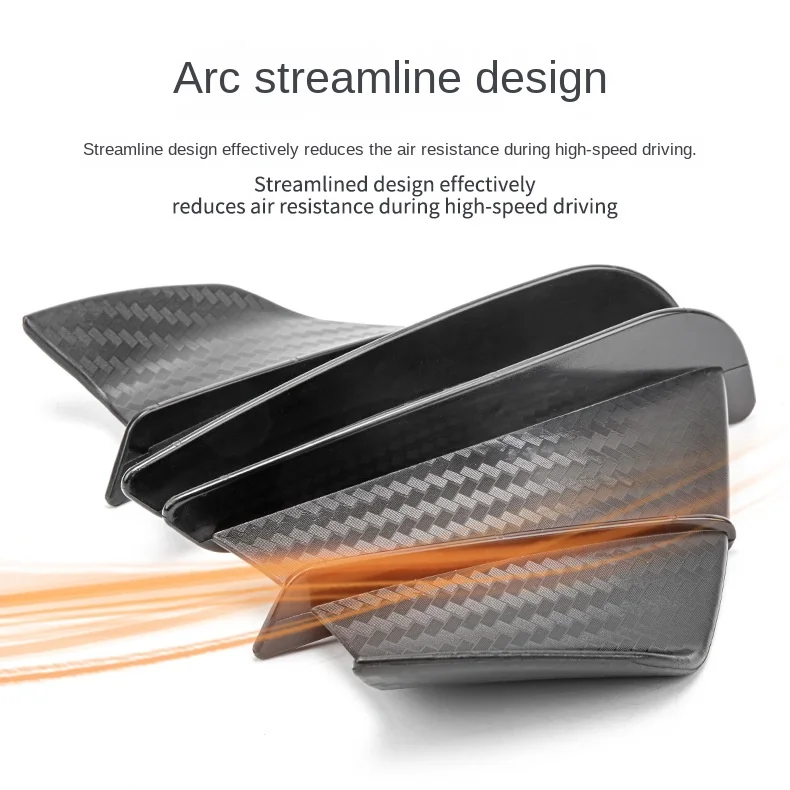The image showcases a highly detailed, 3D-rendered tail fin modification designed for automobiles, prominently titled "Arc Streamline Design" in bold black text at the top. Underneath, it emphasizes twice—once in large print and once in smaller print—the efficiency of the streamline design in reducing air resistance during high-speed driving. The silver tail fin device features a sleek metallic finish, composed of strips of metal with two centrally positioned blades. Both the top and bottom sections are adorned with a checkered pattern of darker and lighter diagonal rectangles, giving it a sophisticated, high-tech appearance. The design is complemented by a vivid orange streak, simulating airflow and flames, which visually demonstrates the aerodynamic benefits. The entire piece is presented on a white background, further accentuating its clean lines and futuristic aesthetic, and appears to be made from a high-quality, possibly 3D-printed, carbon composite material.